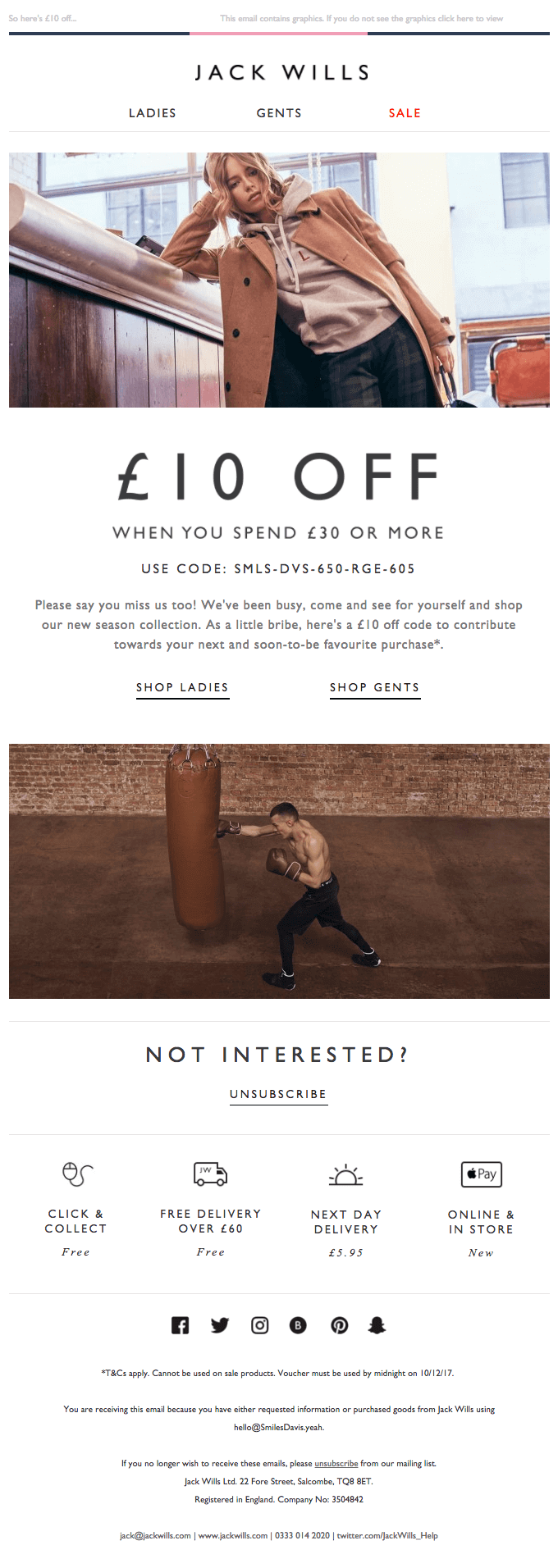The mobile screenshot showcases the shopping website "Jack Willis." At the top, the brand name "Jack Willis" is prominently displayed. Beneath it, there are three key categories: "Ladies," "Gents," and "Sale." The "Sale" section is highlighted in red typeset, drawing attention.

Under these headings, a horizontally oriented photograph features a stylish woman leaning on a counter. She is dressed in plaid pants, a hoodie, and a beige coat, and she holds a handbag in her left hand while looking directly at the camera. Below this image, there is large text stating "£10 off" with a smaller note indicating the offer applies when spending £30 or more, along with a promotional code.

Further down, there are headings for "Shop Ladies" and "Shop Gents," followed by a sepia-toned photograph of a muscular man boxing. He is depicted hitting a large weight suspended from the ceiling with a spread-legged stance. The text beneath this image reads "Not Interested," alongside an underlined "Unsubscribe" link.

Below this, various icons and text indicate extra services: "Click and Collect," "Free Delivery over £60," "Next Day Delivery," and availability "Online and In-Store." Finally, there are icons for six social media platforms and additional, barely legible, small text.